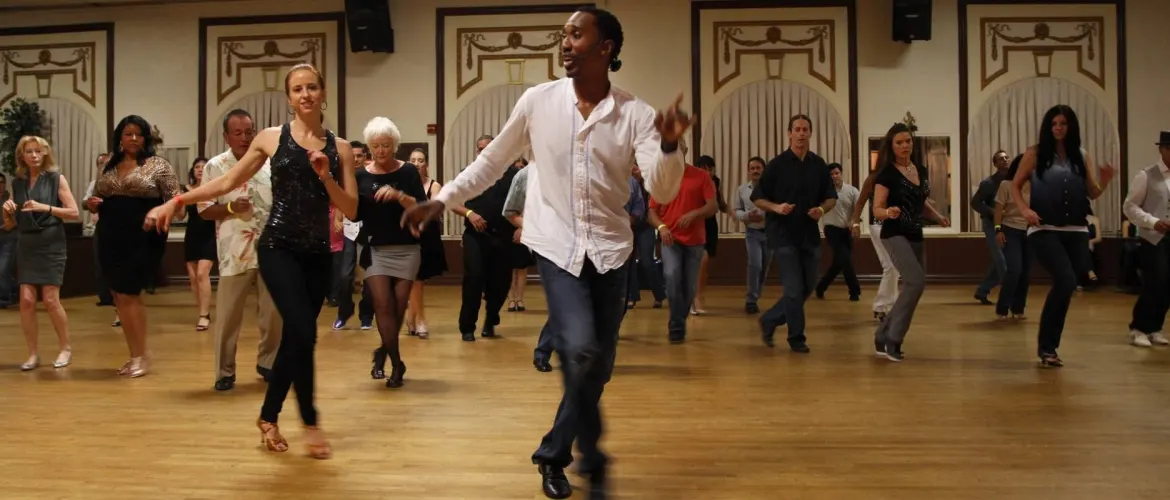This photograph captures a coordinated dance class in a large, well-lit dance room with a light wooden floor and intricately designed white and brown walls featuring square and circular patterns. At the forefront stands the instructor, a dark-skinned male, dressed in a white long-sleeved button-up shirt, blue jeans, and black shoes, with his hair styled in a bun. His stance, with legs crossed and a dynamic arm position—left finger pointing, right arm down—suggests he is guiding the class through a move. To either side and slightly behind him, over twenty dancers are arranged in three rows. The dancers, a mix of varying ages including some elderly participants, are captured mid-step; their legs crossed behind their front leg and arms raised, indicating they are in motion, possibly engaging in a western-style line dance. The group’s attire is predominantly casual, featuring jeans and comfortable shirts, with a few women in skirts or dresses, creating a cohesive yet varied visual of synchronized movement.